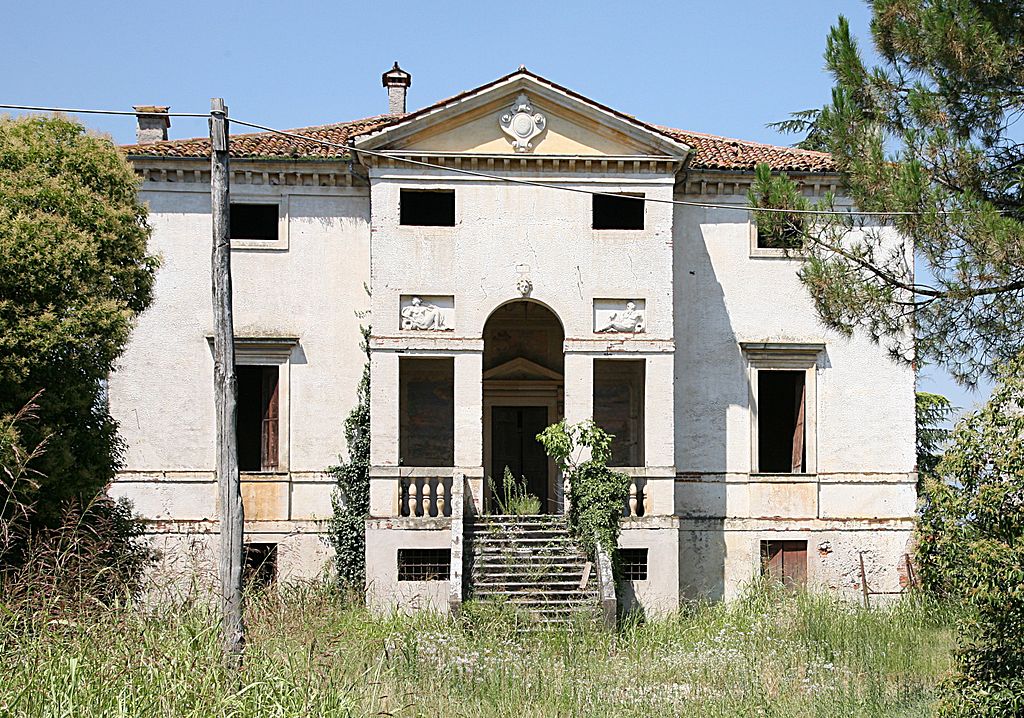This image captures a neglected, three-story colonial-style home constructed from light cream, possibly white stone, and topped with a red tile roof featuring a chimney. The building is architecturally rich, showcasing a prominent arch doorway flanked by sculpted inlets containing personified statues, and crowned by a sculpted head above the arch. The front facade displays square windows, although many are now merely open voids, reflecting the building's state of disrepair. The structure features an ornate pediment with dentil moldings beneath the eaves. The centerpiece of the home projects forward, with the left and right sections recessed. Stairs ascend to the small porch and arched entryway, bordered by banisters and supported by concrete columns. Overgrown grass, trees, and assorted shrubbery envelop the property, with weeds infiltrating the steps and porch, hinting at the building's abandoned state. The overall neglect is palpable, with plants sprouting from the foundation and roof damage evident.